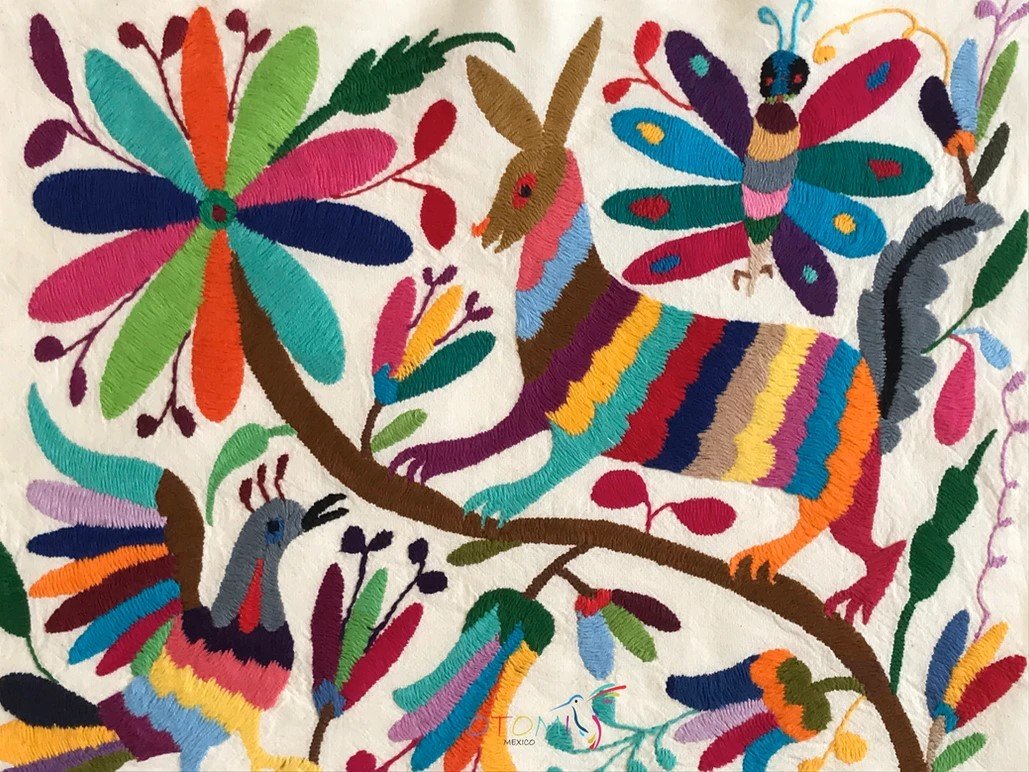This vibrant and intricately designed fabric artwork features a white backdrop and is filled with a dazzling array of colors including pink, green, turquoise, gray, purple, orange, red, and blue. In a landscape layout, it displays multiple stitched elements that depict scenes of outdoor life. A prominent flower with a brown stem and multi-colored petals—turquoise, dark blue, green, and orange—extends from the lower right to the upper left corner, boasting a green center. Perched on the flower is a whimsical bunny with a brown head, embellished in stripes of pink, blue, brown, purple, yellow, green, and red. Above this bunny, a butterfly with a black head has its wings stitched in various colors, adding to the vibrant tapestry. In the lower left corner sits a bird with a gray head, similarly adorned with colorful, striped yarn. Additionally, a caterpillar can be found stitched into the upper right corner of the fabric. The overall piece, with its meticulous stitching and patchwork of colors, evokes the feel of a decorative rug or welcome mat, making it a celebration of nature and color in fabric form.